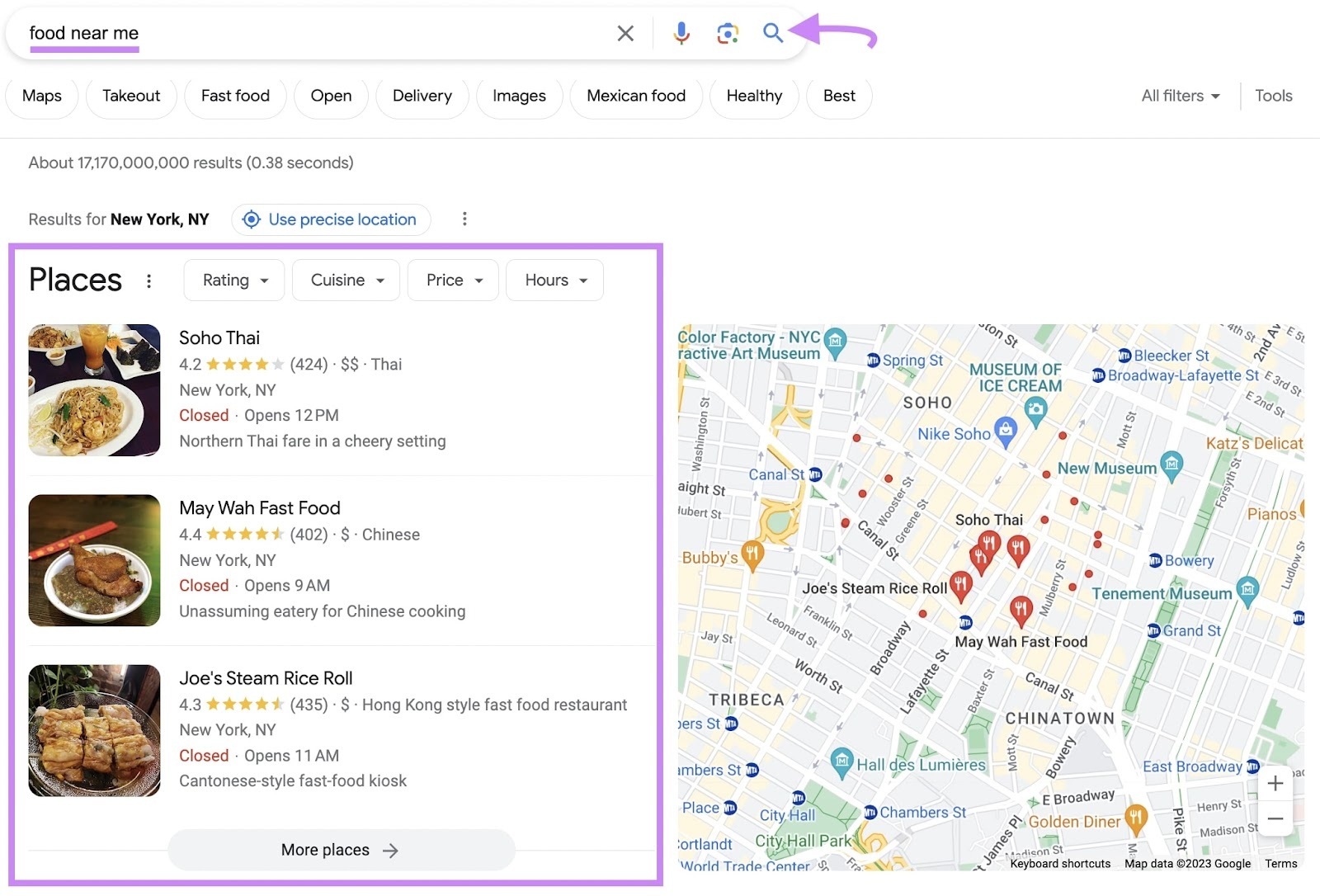In this detailed image, the top section features a search bar with the query "food near me" underlined in purple. The search bar includes icons: an X button, microphone button, camera button, and a magnifying glass search button indicated by a purple arrow. Below the search bar, there is a row of category labels such as "Maps," "Takeout," "Fast Food," "Open Now," "Delivery," "Images," "Mexican Food," "Healthy," and "Best." 

To the far right, there is a "Filter" section labeled "All Filters," with an adjacent "Tools" option. Beneath these labels, the search results indicate approximately 17,170,000,000 results found in 0.38 seconds, followed by a line stating: "Results for New York, New York," with "New York, New York" prominently bolded in black. Right next to it, the text "using precise location" is accompanied by a pinpoint location icon.

The main section is divided into two parts. On the left-hand side, within a purple-outlined box labeled "Places," there are further options for sorting by rating, cuisine, price, and hours. Each category can be clicked to reorder the results accordingly. Below these options, three restaurants are listed, each with corresponding images: 

1. Soho Thai
2. My Wok Fast Food
3. Joe's Steamed Rice Roll

On the right-hand side, a map displays colored pins—red, blue, and orange—indicating the locations of these restaurants.